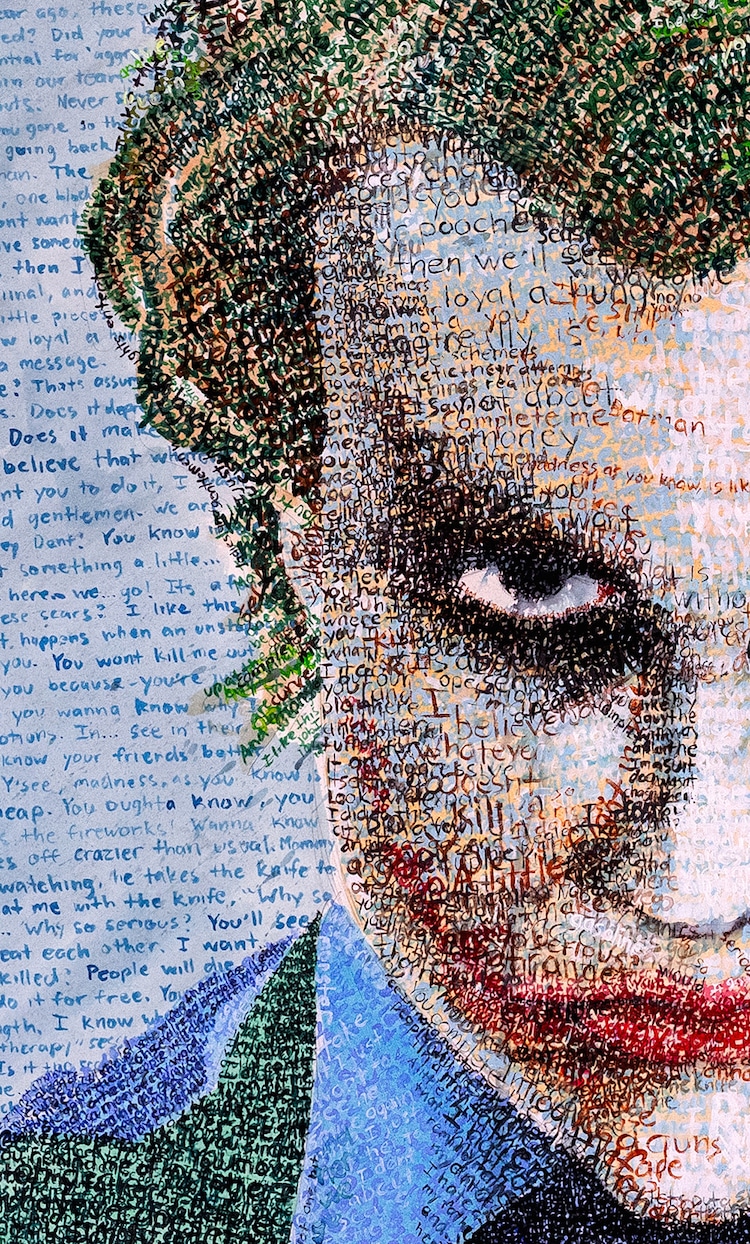This image is an intricate mixed media artwork featuring a highly detailed depiction of the Joker from the Batman series, specifically inspired by Heath Ledger's iconic portrayal. The Joker's face is formed entirely through an array of colored text that artistically shapes his features. His eyes are marked by distinctive black rings, and his lips are an elongated, vivid red, extending up his cheeks. The left side of the portrait is unfinished, giving a sense of incompleteness which underscores the chaotic nature of the character. His hair is a mix of brown and green, scraggly and unkempt, and what little is visible of his blue and green clothing extends slightly to the left.

The background is saturated with seemingly disorganized, multicolored text, contributing to a psychotic and unsettling ambiance. Key phrases embedded within this chaotic typography include "you want to kill me," "you wanna know," and the infamous "why so serious?" These snippets capture the Joker's menacing and unpredictable persona. The techniques used in the artwork include pen, ink, paint, pastels, colored pencils, and markers, all contributing to the textured, layered visual effect that is both intriguing and disturbing.